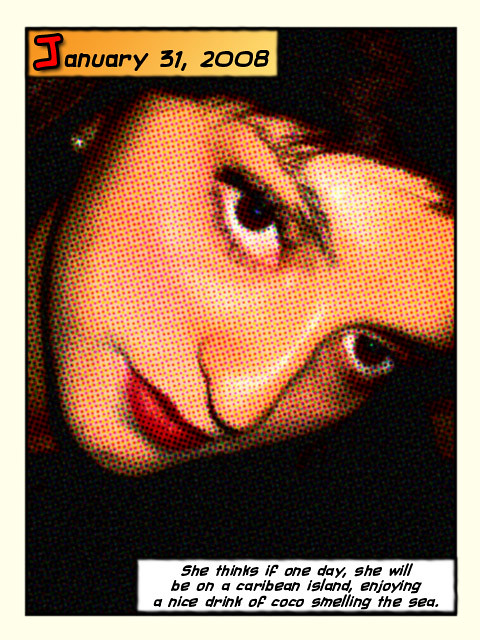This image features a pixelated, almost cartoon-like portrayal of a woman's face, zoomed in and treated with a comic book filter that exhibits colorful printing dots. Her head is tilted down and slightly towards the left, adorned with short dark brown hair that falls just above her eyebrows. She has strikingly shiny red lips and distinctively brown eyes; the eye on top features a blue dot in the center, while the other eye sports a green dot in the center. She is also wearing a diamond-like sparkling earring in her left ear. An orange square with a red "J" and black text reads "January 31, 2008," positioned offset to the left at the top. At the bottom of the image, there is a white rectangular box with black text that reads, "She thinks if one day she will be on a Caribbean island enjoying a nice drink of cocoa smelling the sea." The background is predominantly dark and shadowy, emphasizing the complex and colorful elements of the woman's face.